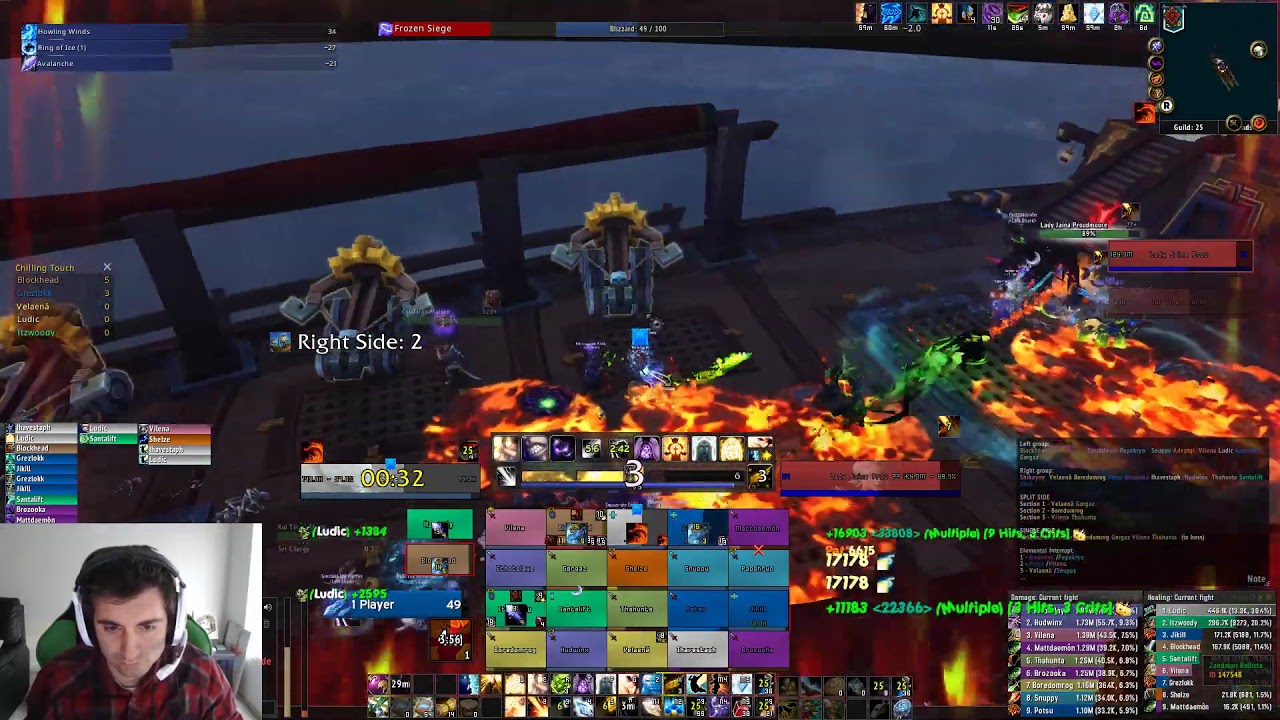The image is a vivid and chaotic screenshot of a live-streamed video game featuring a prominent streamer. Located in the bottom left corner, the streamer is a man wearing a black and red plaid shirt, seated in a green-backed chair with large white over-ear headphones that have an attached microphone on his left side. The background reveals a white room with another black chair and a window.

The game scene itself is set on a large platform that appears to be the deck of a ship, teeming with intense action and fiery battles. Players are launching attacks on each other using various colored flames—orange and green are notably mentioned. The front of the ship is armed with three lined-up cannons or guns, adding to the chaotic warfare scene. Fire and lava spread across the platform amidst a myriad of vibrant colors, ranging from pink and orange to yellow, blue, and purple. Numerous boxes with text and tiny image icons populate the lower part of the screen, likely displaying player information and stats. The game's complexity and intensity suggest a challenging and dynamic battle environment, captivating not just the streamer but also the engaged viewers in the live chat below.